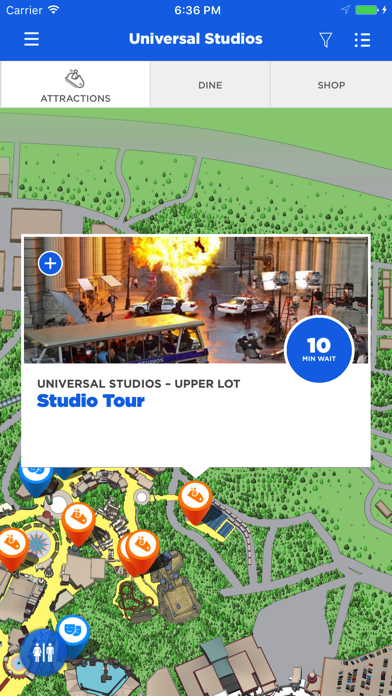This screenshot, captured on a smartphone at 6:36 p.m., displays the Universal Studios app. The phone’s status bar reveals the carrier signal, a connected Wi-Fi symbol, and a fully charged battery with the device plugged in. The app's interface showcases the title "Universal Studios" prominently at the top, beneath which are three clickable tabs: Attractions, Dine, and Shop. With the Attractions tab selected, the main content of the screenshot is a detailed map of Universal Studios.

The map features a green background with pathways highlighted in gray and yellow shades. Various attraction icons are scattered across the map: orange rollercoaster symbols representing thrill rides and light blue theater mask icons indicating shows or performances. Notably, at the bottom left of the map is a circular restroom sign.

A pop-up window highlights the "Universal Studios Upper Lot Studio Tour" attraction. This window, with a white background, provides additional information: a blue circle indicates a 10-minute wait time, accompanied by a background photo of the Studio Tour. The map's intricate details and the clear labeling of attractions make it an essential tool for navigating Universal Studios.